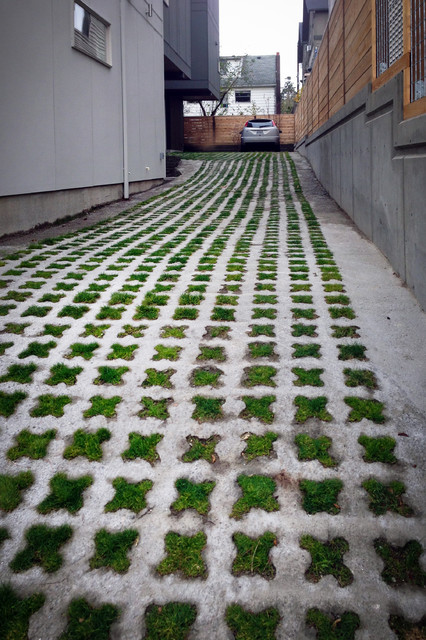The image depicts a decorative driveway or alleyway nestled between two buildings. The path is distinctive, adorned with a pattern of small green crosses every four inches, creating neat rows that continue along the length of the driveway, giving it an ornamental and almost carpet-like appearance. On the right, a taller wooden structure painted in brown and gray stands, while on the left, part of a gray building is visible, featuring a single window. This driveway, set with narrow cement borders on either side of the green section, leads to a gray car parked under an overhang or shed that has enough space to accommodate two vehicles. In the background, a brown privacy fence marks the end of the path, with a white house and gray roof seen beyond it, and a sliver of sky peeking through the top of the scene.